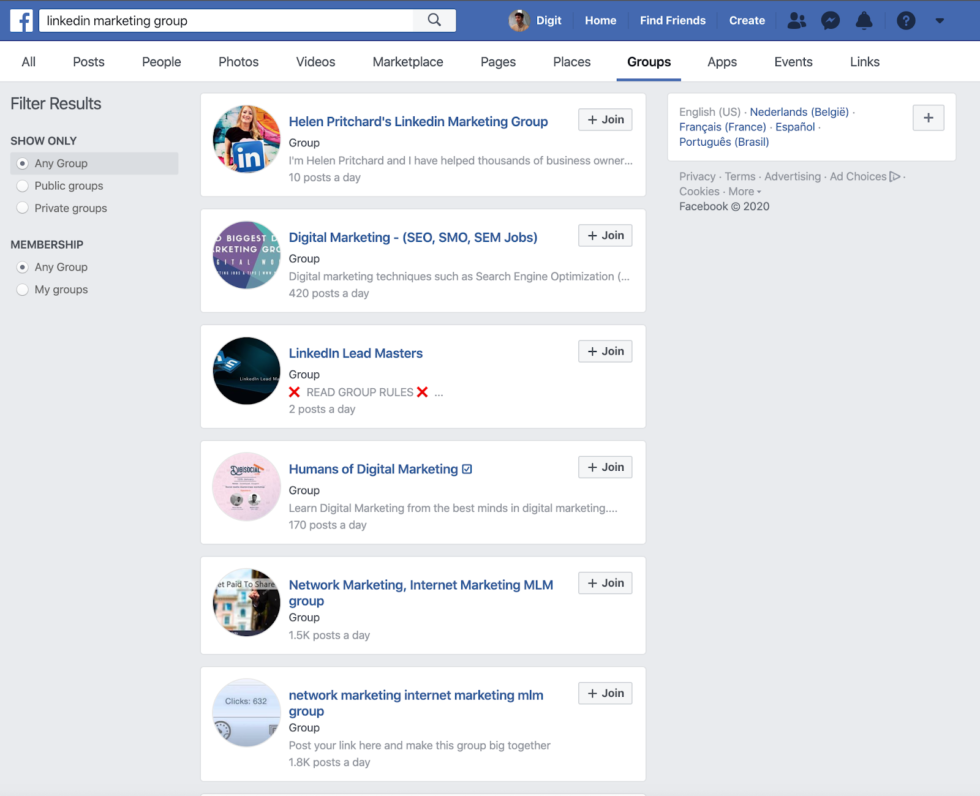This image is a detailed screenshot of a Facebook application interface, likely taken on a computer. The photo is roughly square-shaped, featuring a prominent blue horizontal border at the top. On the left side of this border, there is a white box containing the iconic blue "F" symbol of Facebook. Adjacent to this is a white search bar displaying the text "LinkedIn marketing group," accompanied by a magnifying glass search icon.

To the right of the search bar, there is a small circular avatar, difficult to discern due to the zoom level, but it seems to depict a male individual wearing a pink shirt. Flanking the avatar are several white text labels, including "digit," "home," "find friends," "create," followed by gray icons representing "people," "messages," "notifications," and "questions."

Beneath this blue border, another white horizontal border appears, containing several tabs: "all posts," "people," "photos," "videos," "marketplace," "pages," "places," "groups," "apps," "events," and "links." The "groups" tab is highlighted with a blue underline, indicating it is the currently selected category.

Below this header, the interface displays multiple search results related to LinkedIn marketing groups. The listed groups include "Helen Pritchard's LinkedIn marketing group," "digital marketing," "LinkedIn leadmasters," "humans of digital marketing," "network marketing," and others, with some groups repeating to emphasize their relevance.

On the left side, there is a filtering panel featuring "show only" and "membership" options, which include three choices under "show only" and two under "membership." On the right side, a white box labeled "English" is visible, offering an option to select the desired language for search results.